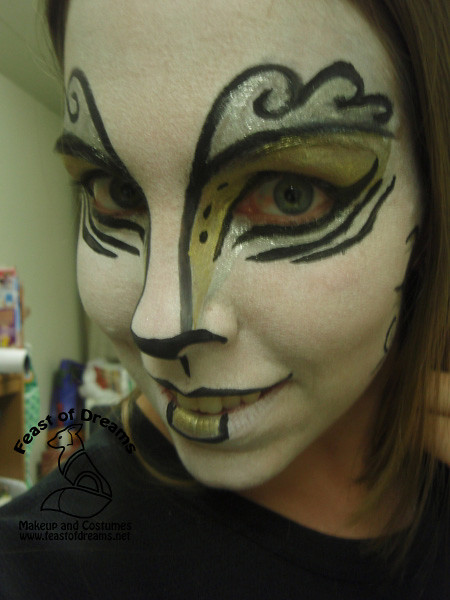A super close-up selfie of a woman with a dark brown hair and elaborately painted face, which resembles an animal. Her face is covered with a very white base and intricate black ink patterns. Her eyes are surrounded by cloud-like eyebrows and cat-like stripes, extending from her eyebrows down her nose, with additional black dots and lines. Her nose is accented with black lines, further enhancing the animalistic look, and her lips are painted white with black outlines and small black lines on the bottom lip. She is smiling and showing her teeth, and she is wearing a black t-shirt. In the background, there are shelves and a drawing of a fox on the left side of the image with the text "Feast of Dreams, Makeup and Costume" and a website.